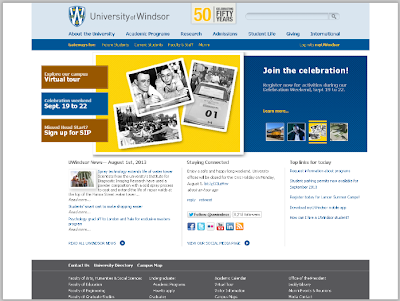Screenshot of the University of Windsor's Website Celebrating 50 Years

The screenshot captures the University of Windsor’s website, commemorating its 50th anniversary. The website features a clean, white background framed by white borders on the left and right sides. At the top, there is a blue banner with the university’s logo prominently displayed—a stylized 'W' inside a shield-like icon. Accompanying the logo, text reads "University of Windsor 50" and "50 years", symbolizing the milestone celebration.

Adjacent to the logo, there is a search bar along with several navigation links including "About the University", "Academic Programs", "Research", "Admissions", "Student Life", "Giving", and "International". The print is small, making some text hard to discern.

On the left side of the page, various informational boxes are displayed. One brown box invites visitors to "Explore Our Campus" via a virtual tour. Another blue box highlights important dates: "September 19-22," alongside an apparent invitation to sign up for SIP. A yellow box features three black and white, Polaroid-style photographs of people in a vehicle, contributing a nostalgic touch.

To the right, a bold blue box with white text encourages users to "Join the Celebration," with an accompanying yellow button labeled "Click More." Below this call-to-action, there’s additional text in blue and black on a white background, although much of it is difficult to read due to the small font size.

At the bottom, a gray border contains contact information and social media icons for Facebook, LinkedIn, YouTube, and a podcast/listen icon, enhancing connectivity.

Overall, the webpage effectively combines functional navigation with celebratory elements to mark the University of Windsor’s significant anniversary.